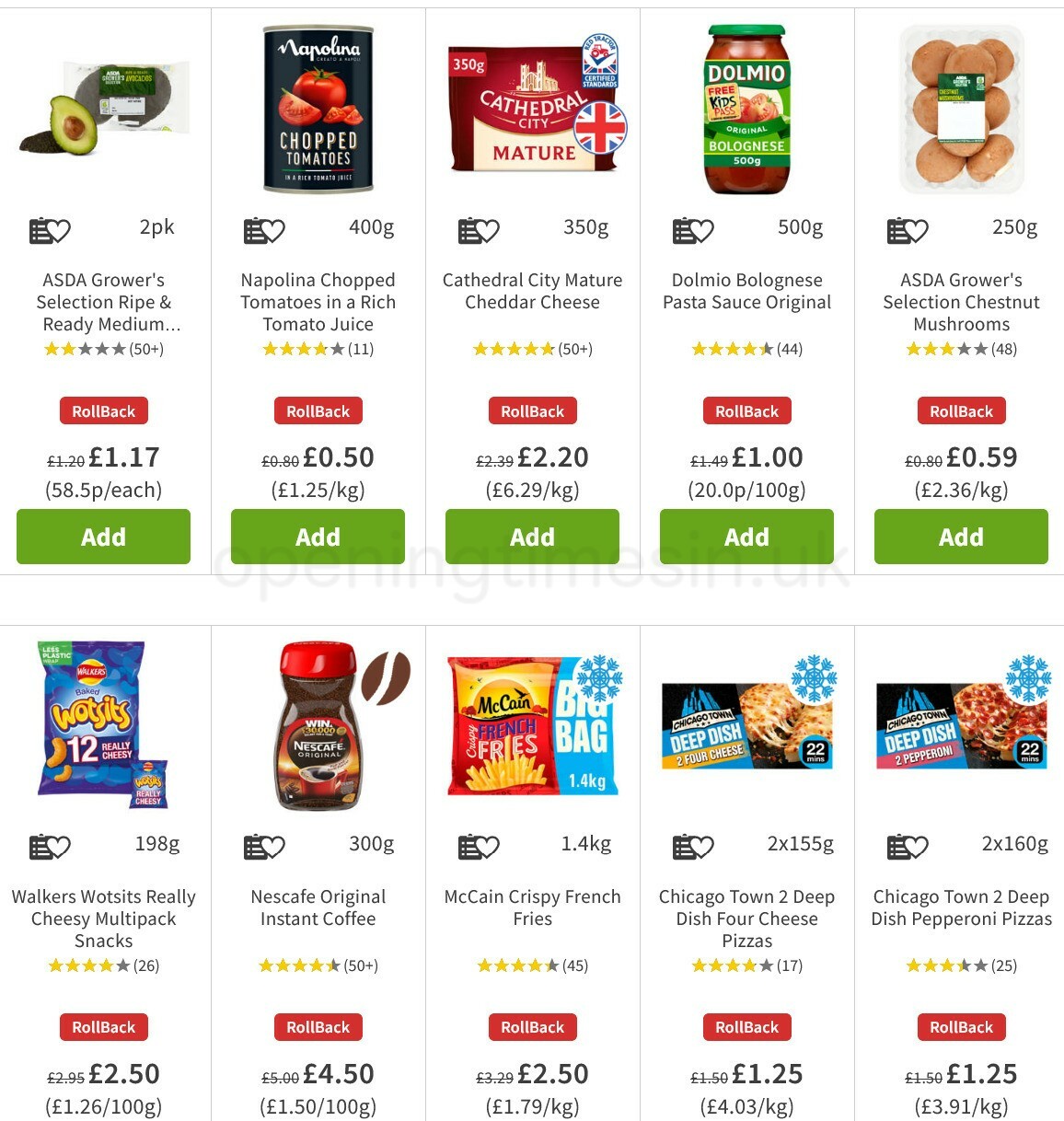The webpage displayed showcases a variety of stock items alongside their prices. Featured prominently is ASDA's Grower's Selection of ripe and ready medium tomatoes, presented next to Napolina's chopped tomatoes immersed in rich tomato juice. The selection continues with Cathedral City's mature Cheddar cheese, followed by Dolmio's Bolognese pasta sauce in its original flavor. Also included are ASDA Grower's Selection chestnut mushrooms, and Walker's Wotsits Really Cheesy multi-pack snacks. The range extends to Nescafé Original instant coffee, McCain Crispy French Fries, and Chicago Town Deep Dish pizzas. Each item is clearly labeled with its corresponding price, offering a comprehensive snapshot of available groceries.